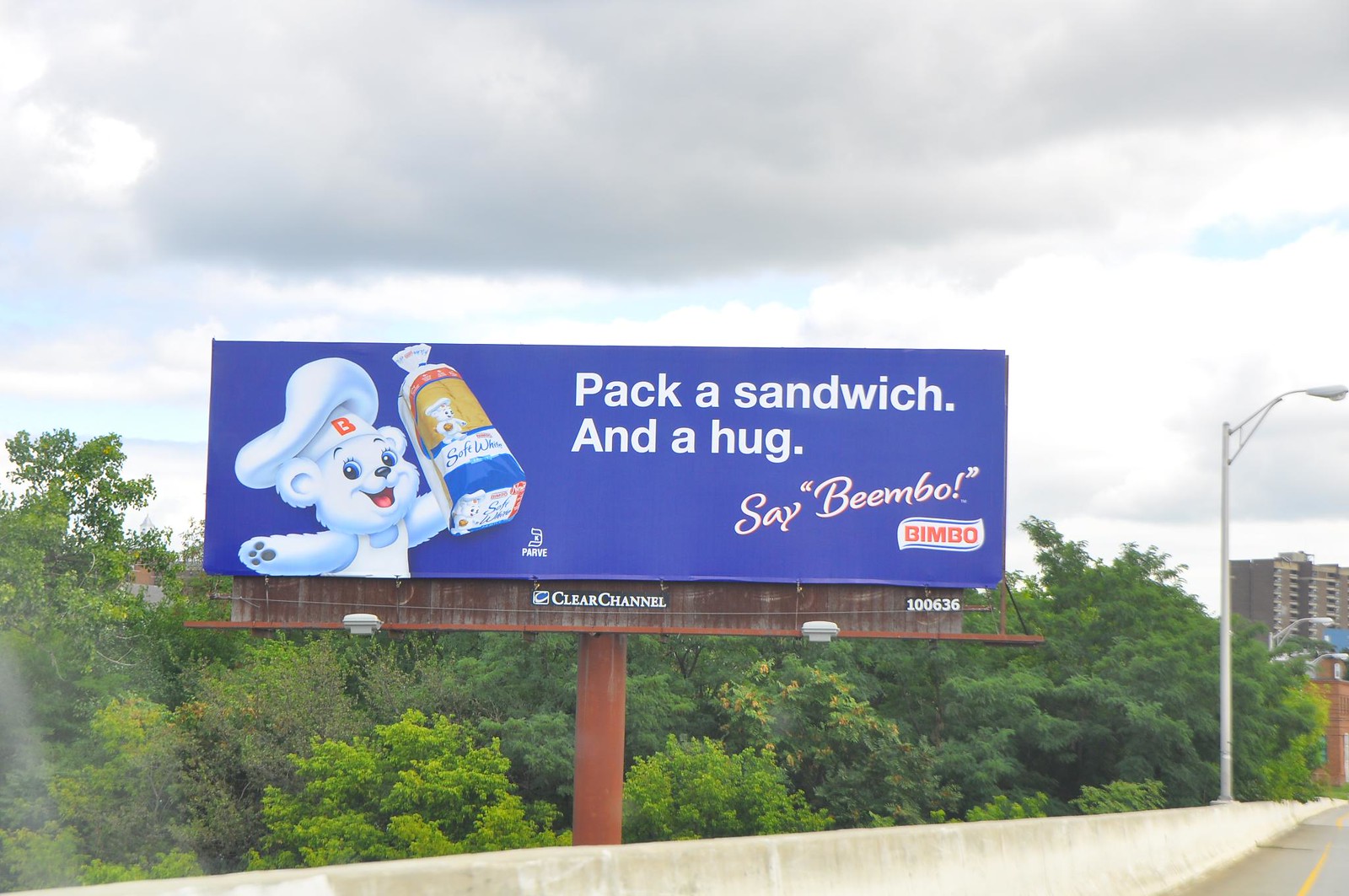This image depicts a large billboard prominently placed along a freeway, supported by a massive metal pole. The billboard's dimensions are approximately four times wider than it is tall, and it features a bright blue background. Central to the advertisement is a cheerful white bear wearing a chef's hat adorned with a red "B" and a cut-off white t-shirt. The bear is smiling and holding a loaf of bread in its left hand, which also displays the bear's image surrounded by a yellow background and illegible blue cursive writing. 

To the right of the bear, the sign reads in white lettering, “Pack a sandwich and a hug, says Bimbo,” with "B-I-M-B-O" clearly printed below. Below the sign is a label for the advertising company, Clear Channel. The setting appears to be urban or suburban with a high-rise building visible in the background, along with tall streetlights, and a dense line of trees. A concrete barrier runs along the bottom of the image, separating the freeway visible on the right from other roads or areas. The sky is a mix of dark clouds and patches of blue, giving the scene a dynamic and slightly overcast appearance.